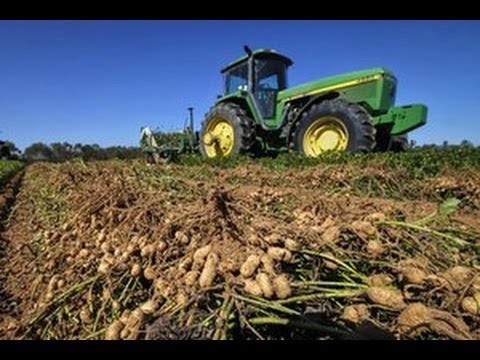The photograph captures a vibrant scene on a field with a centerpiece of a large, green John Deere tractor. The camera angle is uniquely low, as if placed in a ditch, providing an upward-looking perspective of the imposing tractor. The tractor is characterized by its massive black tires with yellow hubcaps, a defining green engine at the front, and a glass enclosure for the operator at the back. Behind the tractor is a plow, actively tilling the soil.

In the foreground, rows of potatoes are partially unearthed, their dirt-covered forms surrounded by green stalks and grass. The soil is rich and dark, with visible roots intertwined beneath the surface. The background offers a serene vista of a blue sky, medium-sized darker green trees on the left, and a distant farmhouse on the right. Shadows cast by the sun highlight the textures and shapes, particularly apparent on the potatoes spread throughout the image. The photograph frames the scene with a thin black border, focusing attention on this harmonious blend of agriculture and machinery.